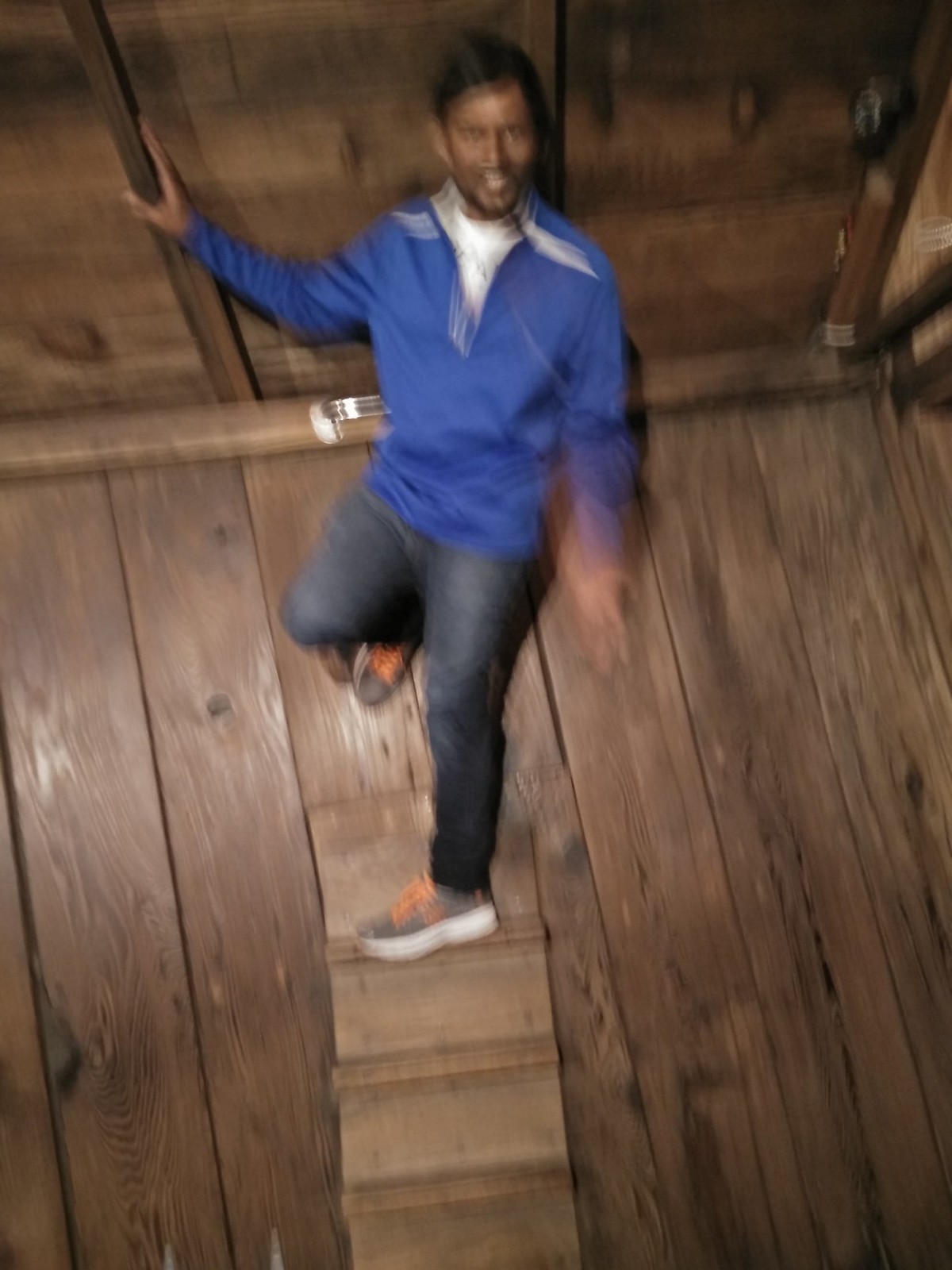In this image, a man is captured mid-action in a slightly blurry, out-of-focus photograph. He appears to be inside a rustic cabin, evident from the wooden walls and ceiling surrounding him. The man has ascended a small ladder and is now gripping the ceiling for support, having turned around to face the camera. His left hand is motion-blurred, while his right hand is firmly holding onto the ceiling. He is dressed casually in blue jeans, a blue jacket over a white shirt, and blue sneakers with striking orange laces. The man, who has dark hair, is staring directly into the camera lens with a slightly elevated position, suggesting the camera was angled slightly below him.